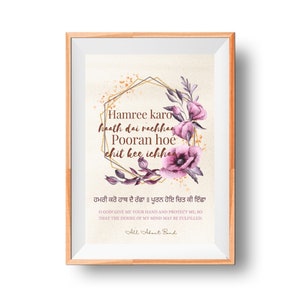The image depicts a framed print with a light wooden frame and a white inner border. Within the frame, the print features a central text area, bordered by a delicate floral design comprised of purple flowers and dark leaves predominantly along the right side. The main quote is printed on off-white paper, and below it, there is additional, smaller text that is difficult to read. Surrounding the central quote is a black border line, and near the bottom center of the print, a small, barely legible signature is visible. The frame casts a subtle shadow to the right and at the bottom on the otherwise white background, suggesting it is slightly elevated from the surface it rests on. This neat and aesthetically pleasing decoration seems like it would be an ideal addition to a home, potentially measuring around 12 inches in height.